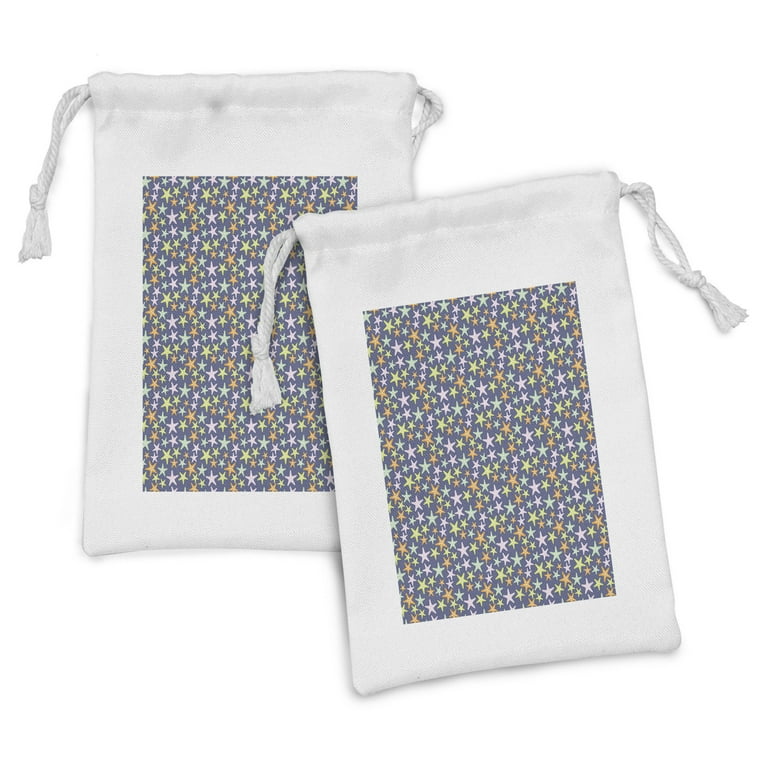In the image, we see two small, white cloth pouches, each adorned with a design featuring many stars. The stars, rendered in various colors including white, pale yellow, light orange, and gray, are set against a dark grayish-blue rectangular background at the center of each pouch. Both pouches have a closure mechanism involving white tassels at the top, which can be pulled away from each other to secure the contents inside. The background of the image is white, and one pouch is slightly placed on top of the other. These decorative pouches appear suitable for storing small items like jewelry or dice.